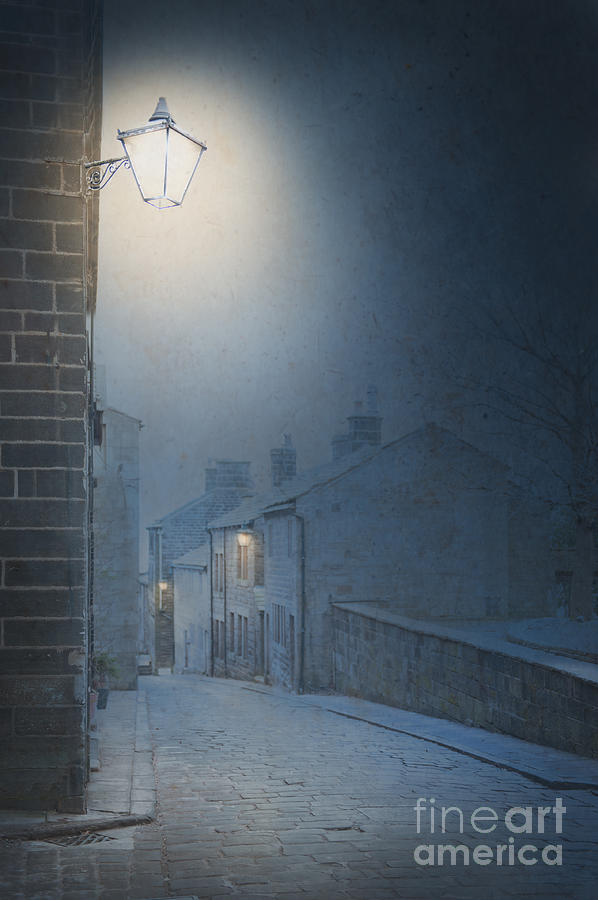The vertically aligned rectangular image resembles a sketch and portrays a Victorian cobbled street at night during winter. On the left side, a brown brick building with a lit lantern attached to it emits a yellow glow. The area behind the lantern is brightened by this light, in contrast with the dark nighttime sky that envelops the top portion of the image. On the right side, thin, leafless tree branches extend into the frame, possibly with some leaves blowing and tiny dots scattered throughout the picture, hinting at falling snow or fog. Below the tree branches, a narrow cobbled pathway can be seen leading between a retaining wall and a lineup of white buildings that appear to be either apartments or houses. The center building in the background sports a lit window with a light above it, casting a misty hue. Additional details include chimneys topping the buildings, reinforcing the Victorian ambiance. At the bottom right corner, the word "Fine Art America" is inscribed in gray letters.